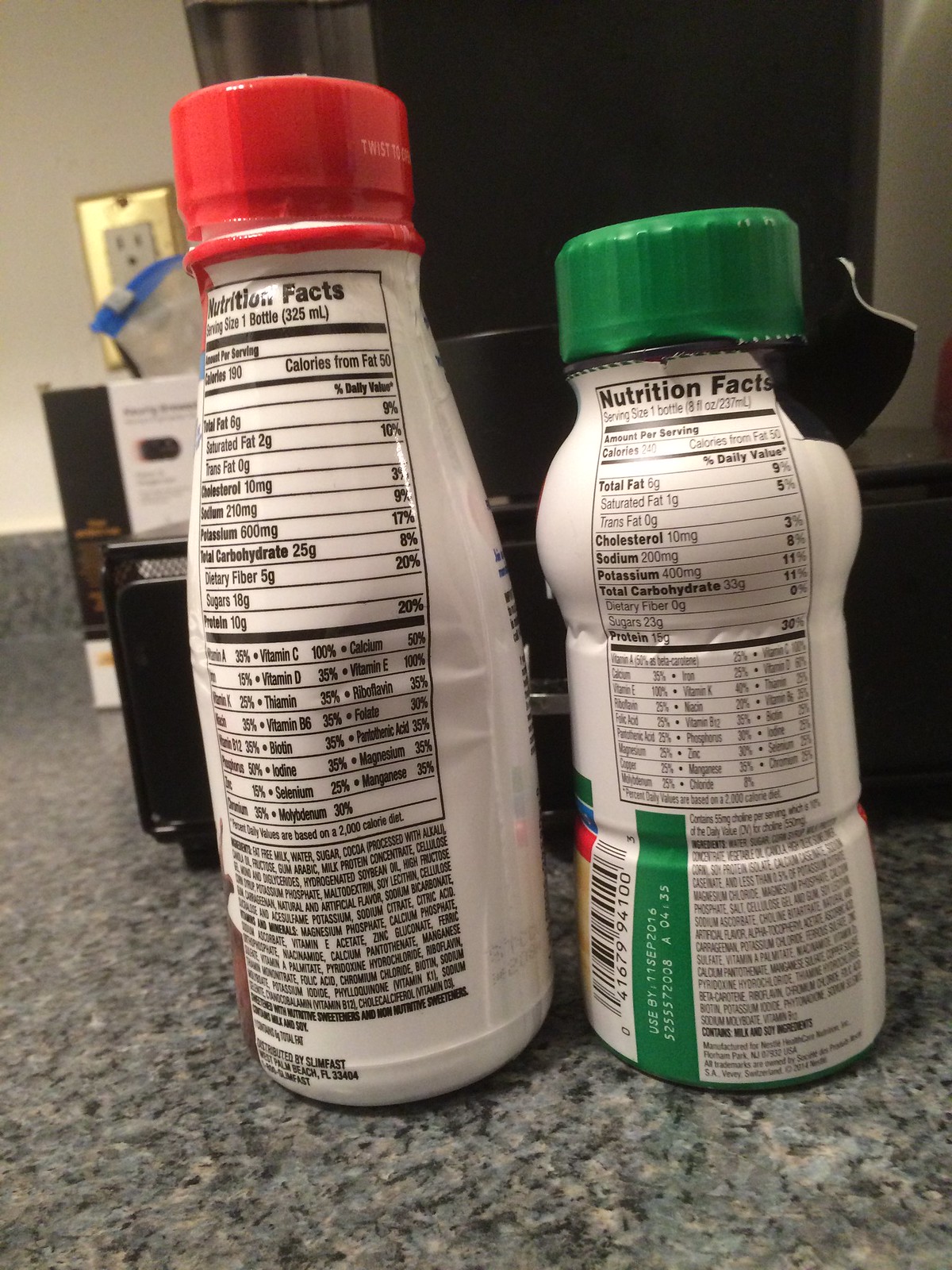This is a highly detailed color photograph of two plastic beverage bottles placed side by side on a gray granite countertop with black and white specks. Both bottles are turned with their backs facing the camera, displaying their nutritional information. The taller bottle on the left has a red cap and a cylindrical shape that narrows towards the top. The nutrition label denotes a serving size of one bottle (325 milliliters), containing 190 calories with 50 calories from fat. Specific nutrition details include 6 grams of total fat (9% DV), 2 grams of saturated fat (10% DV), and others like cholesterol, sodium, potassium, carbohydrates, dietary fiber, sugars, protein, and various vitamins. 

The shorter bottle on the right features a green cap and a wider shape that narrows towards the center then widens again at the top before tapering near the neck. It has an 8 fluid ounce (237 milliliters) serving size with 240 calories per bottle, including 50 calories from fat. It lists details like 6 grams of total fat (9% DV), 1 gram of saturated fat (5% DV), plus cholesterol, sodium, potassium, carbohydrates, dietary fiber, sugars, and protein content, along with additional vitamin information and ingredients at the bottom of the label. Additionally, this bottle has a barcode visible on its left side. 

In the background, there is an indistinguishable black object and a white wall featuring an outlet with a brass switch plate cover.